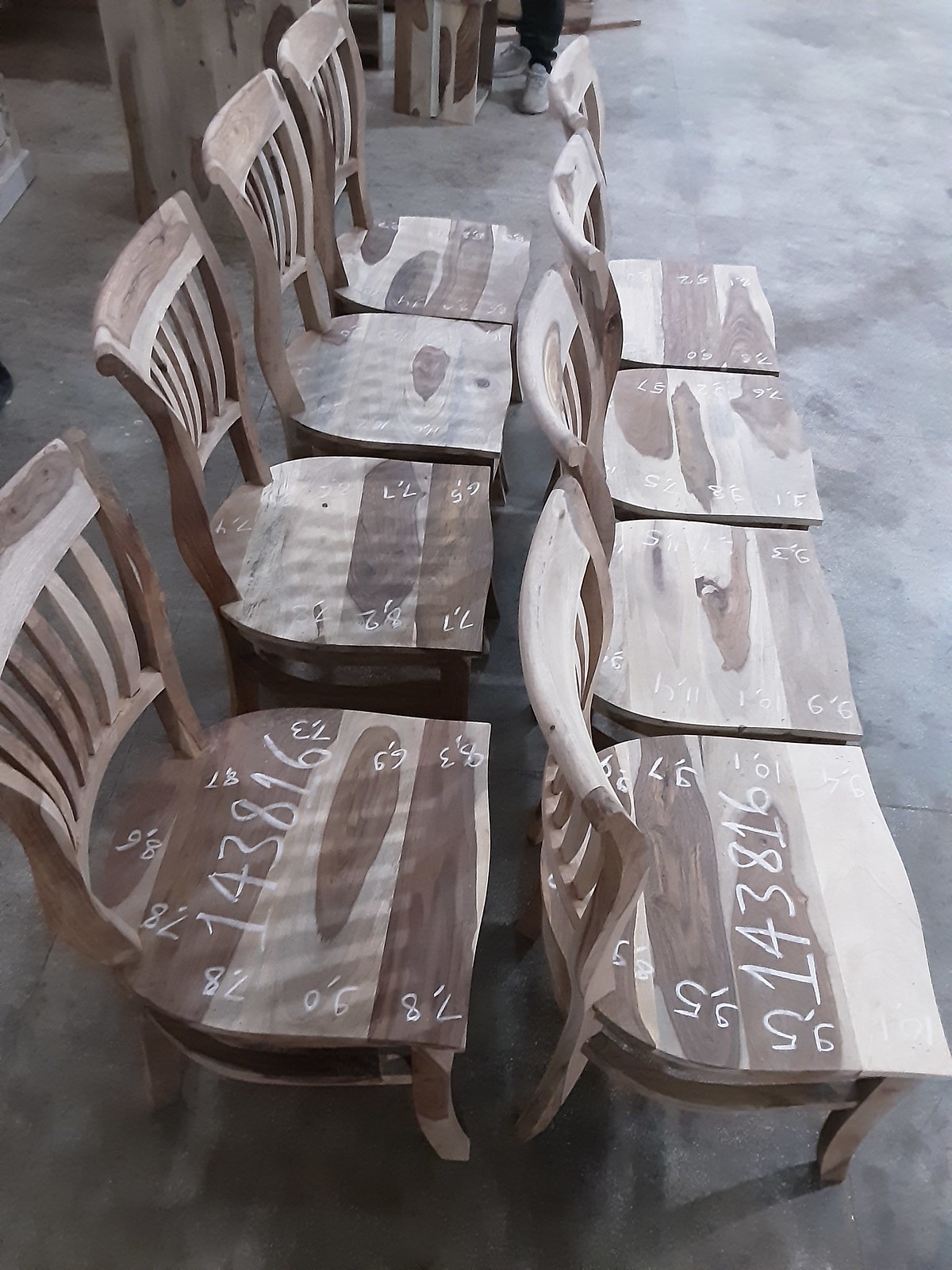This photograph features eight wooden chairs arranged in two parallel rows of four each. The chairs, crafted from a mix of dark and lighter brown wood, are set on a concrete or gray marble floor and exhibit reflections on their surfaces. Various numbers and codes are inscribed on the chairs, suggesting they are in the process of being manufactured or identified for quality control. Particularly, one chair in the foreground has "143816" and "95" prominently marked, with an exception near the end that reads "97." Another chair displays the number sequence "789082788687736983," while a subsequent one is marked "77827774." A person's shoes and the bottoms of their pant legs are visible in the upper part of the image, indicating the presence of a builder or worker. This meticulous arrangement and labeling point to a systematic assembly or inspection process in what appears to be a warehouse setting.